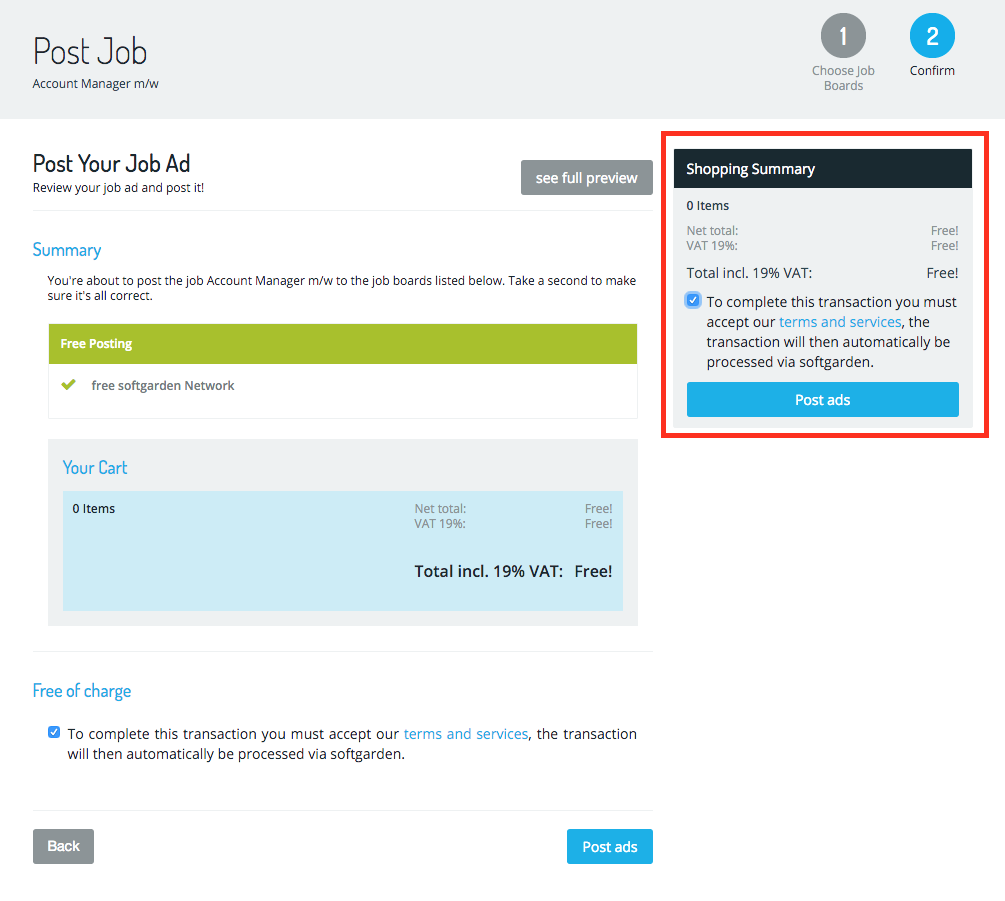This image is a screenshot of a computer monitor displaying an interface for posting a job advertisement. At the top of the screen, there is a thick gray bar with black text on the left reading "Post Job Account Manager M/W." On the right, a gray bubble with a white "1" inside says "Choose Job Boards," and adjacent to it, a blue bubble with a white "2" inside reads "Confirm."

Directly below this bar, on a white background with black text, it instructs users to "Post Your Job Ad, Review Your Job Ad and Post It," followed by a gray box containing "See Full Preview." 

On the right side of the screen, a panel outlined in red provides a "Shopping Summary" detailing "Zero Items," "Net Total," and "VAT 19%." It indicates that the services are "Free," with a note stating "Total Included 19% VAT Free." The panel also contains a blue check box highlighting that "To complete this transaction you must accept our Terms and Services," with "Terms and Services" in blue text. The transaction will be processed via SoftGarden, and there's a blue button labeled "Post Ads."

In the main section of the screen, to the left, there is a green bar with white lettering that reads "Free Posting," and underneath, a white bar with a green check mark indicating "Free SoftGarden Network." Below this, a gray box is overlaid with a blue box. The gray box contains the blue text "Your Cart," while the blue box displays "Zero Items" in black text, along with "Net Total Free," "VAT 19% Free," and "Total Included 19% VAT Free." 

Additionally, there is a statement "Free of Charge" with a blue check mark, mirroring the information in the red-outlined panel. At the bottom left of the screen is a gray "Back" button, and at the bottom right is a blue "Post Ads" button.